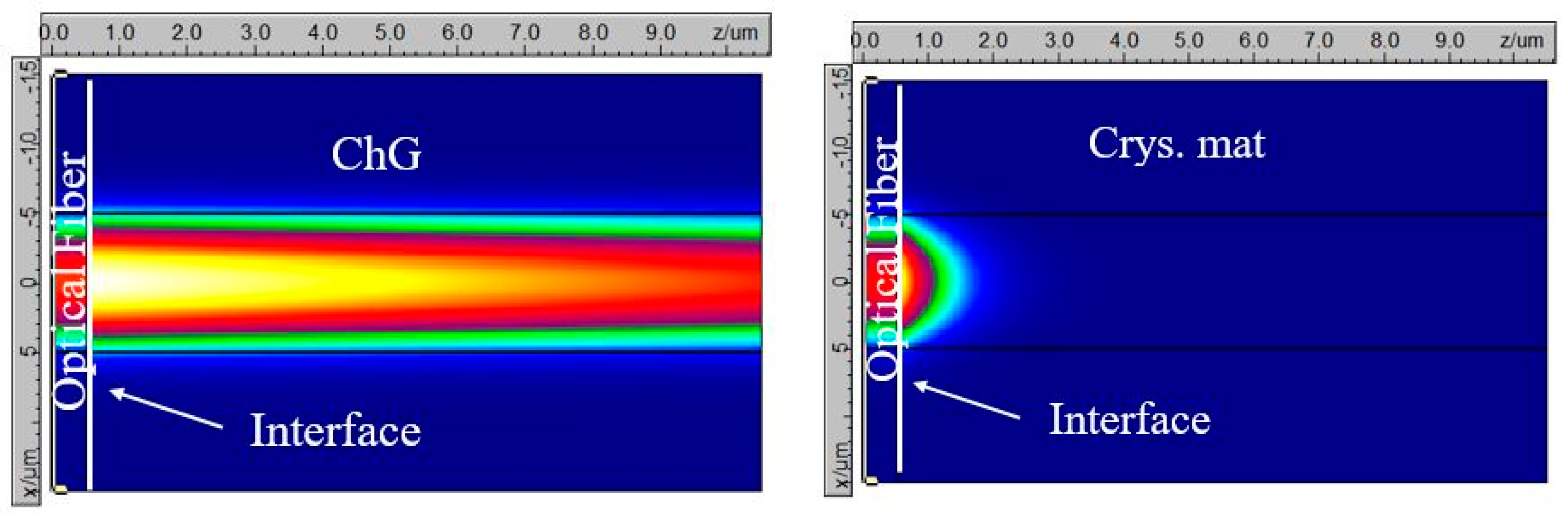This image depicts two side-by-side scientific graphs illustrating heat intensity measurements within an optical fiber system and a crystalline material interface. Both graphs share identical axes: the x-axis ranging from 0.0 to 9.0 (labeled as Z/µm) and the y-axis ranging from -15.0 to 5.0 (labeled as X/µm). The left graph, labeled "CHG" at the top, demonstrates heat transfer from the optical fiber interface into a CHG medium, prominently featuring a spectrum of colors from bright red, orange, yellow, to green. An arrow labeled "interface" points leftwards towards the "optical fiber." The right graph is labeled "CRYS.MAT" at the top, presumably standing for crystalline material, and also designates an "interface" at the bottom. The colorful gradient originating in the first graph traverses into the second, indicating a comparative study of heat transfer properties between the CHG and CRYS.MAT materials.